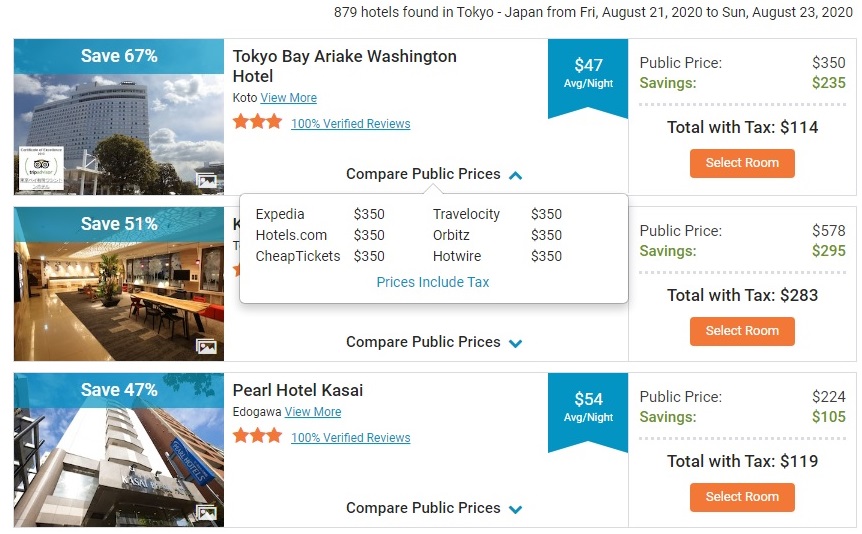Displaying a search result for hotels in Tokyo, Japan, this image features a clear white background with a header indicating "879 hotels found in Tokyo, Japan from Friday, August 21st, 2020 to Sunday, August 23rd, 2020." Below this, on the left side, a vertical column shows three images. 

The bottom image, captioned "saved 67% at the blue sky with clouds," displays a building surrounded by trees. To its right, details about the Tokyo Bay Ariake Washington Hotel, Kodo are provided. It includes:
- A label: "100% verified reviews"
- An average nightly rate: $47
- A public price: $3.50
- Savings: $2.35
- Total with tax: $1.14

Directly beneath this, there is an orange "Select Room" button.

A secondary image below this showcases a room featuring a table, a rug, and a plant. To its right, a pop-up box compares prices from various booking platforms:
- Expedia: $3.50
- Hotels.com: $3.50
- Cheap Tickets: $3.50
- Travelocity: $3.50
- Orbit: $3.50
- Hotwire: $3.50

A blue hyperlink at the bottom of the pop-up box reads "prices include tax."